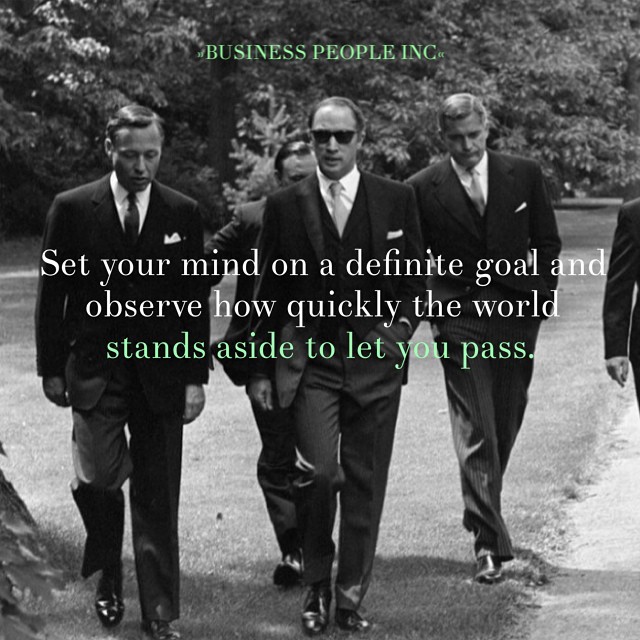This black-and-white photograph captures a striking image of four men dressed in sharp black suits, white button-up shirts, and dark ties, with a hint of another man's arm on the right edge of the frame. The central figure stands out with his black sunglasses and hands in his pockets. The scene unfolds on a grassy area with a dense backdrop of trees, and a dirt path extending to the right. The men, possibly attending a formal event, wear dark vests, fancy leather shoes, and have white handkerchiefs tucked into their jacket pockets. Overlaying the image, green text at the top reads "Business People, Inc." Below, white text states "Set your mind on a definite goal and observe how quickly the world," followed by more green text, "stands aside to let you pass."